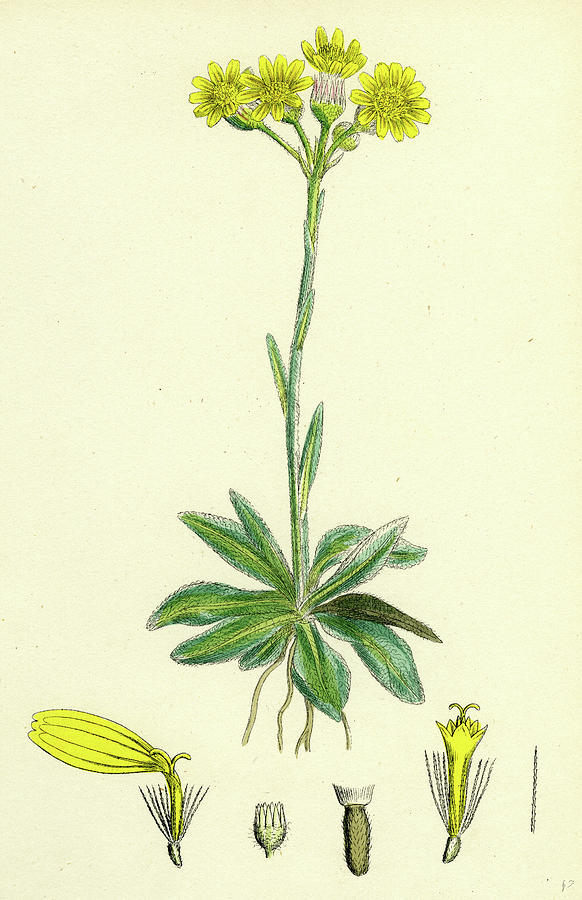This illustration is a meticulously detailed botanical print, possibly a pen and ink drawing enhanced with watercolor, set against a light cream, almost sepia-toned background. Dominating the center, the plant features a long, narrow green stem adorned with leaves near the base and exposed roots, emphasizing its entire structure. Toward the top of the stem, four yellow flowers, which appear to be dandelions, are illustrated in full bloom, displaying their petals, seed pods, and stamens. Below the primary image, the drawing showcases four separate and detailed close-up stages of the flower's development. These sections, rendered with precision, highlight the intricate parts of the blossoms, including bulbs and other elements, contributing to the artwork's educational and aesthetic value. The color palette prominently includes black for the lines, green for the stem and leaves, yellow for the petals, and a touch of brown for certain elements, creating a harmonious and informative depiction of the plant.